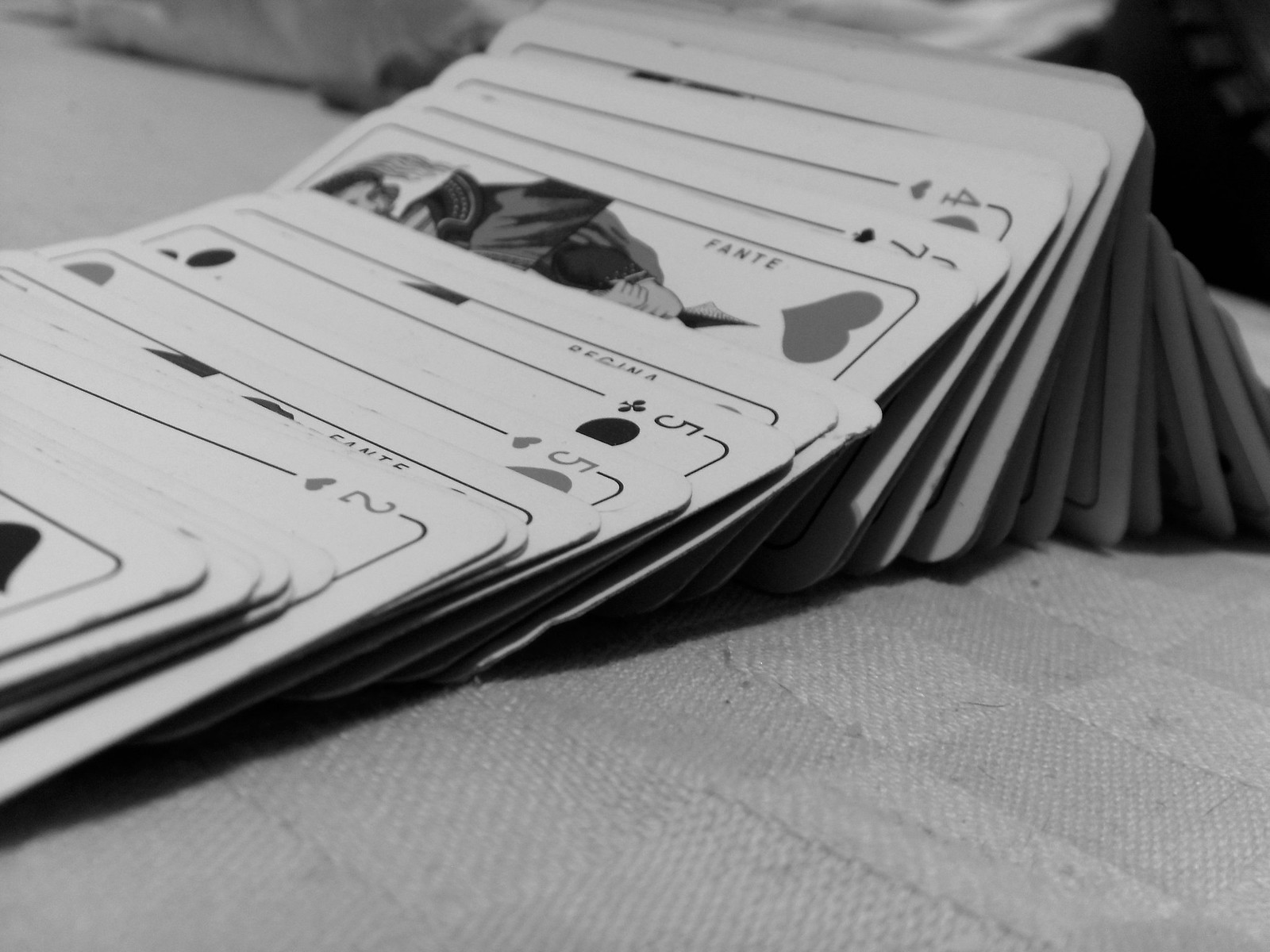This black-and-white photograph features a meticulously arranged deck of cards as its focal point. The background displays a woven blanket with a distinctive checker diagonal pattern, created by a blend of darker and lighter gray threads, interspersed with fine white lines. In the upper right corner, there's a blurry juxtaposition of black and white elements, adding a subtle hint of mystery to the image.

The central subject is a deck of playing cards, artfully leaned against one another to form a delicate peak, from which they cascade downwards. The cards, adorned with heart suits and numerical markings typical of a standard deck, gradually flatten out as they extend towards the edge of the frame, disappearing into the unseen realm beyond the photograph's boundary. The overall composition highlights the intricate details and textures, evoking a sense of both order and dynamic motion.